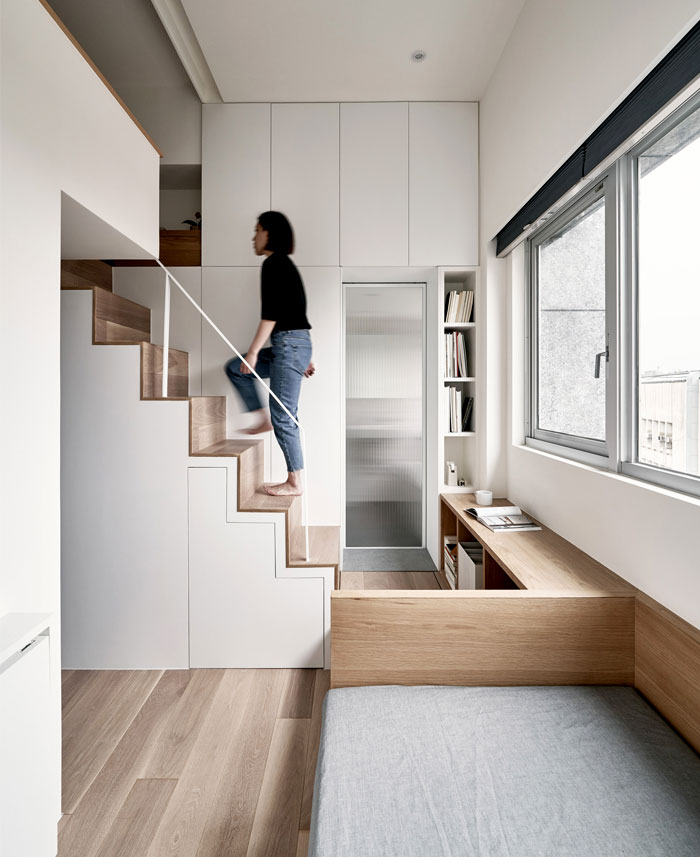The picture depicts a minimalist, modern loft apartment with white walls and unpolished light wood furniture, including a daybed and cabinets. A person, appearing to be an Asian man with short black hair, wearing a black shirt and blue jeans, is captured midway up a staircase with white metal railing, seemingly in motion, suggesting long exposure photography. The apartment features a mix of functional furniture, such as a brown ledge with cupboards underneath, a gray cushioned seating area with a wooden edge, and shelves that blend seamlessly with the aesthetic of the space. Two large windows on the right wall, which overlook other buildings, bring ample light into the room. On the opposite side of the staircase, there are additional white cabinets and a glass door leading to another room. The overall layout and decor emphasize simplicity and a natural wood texture, creating a clean, airy atmosphere.